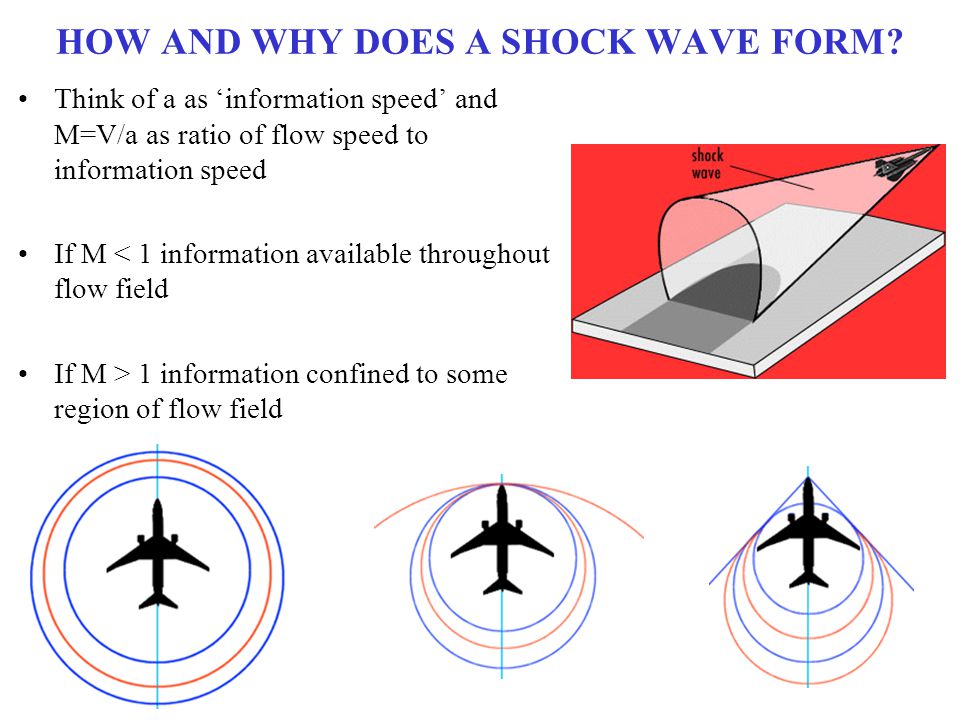The image is an educational illustration on how shock waves are formed. At the top of the page, in bold blue capital letters, is the title: "HOW AND WHY DOES A SHOCK WAVE FORM?" Below the title are three bullet points in black font, aligned left. The first bullet point reads, "Think of A as information speed and M = V/A as ratio of flow speed to information speed." The second bullet point states, "If M < 1, information available throughout flow field." The third bullet point explains, "If M > 1, information confined to some region of flow field."

To the right of these bullet points is a diagram with a red background, showing a red rectangle that illustrates a tunnel with a cone shape pointing towards the center. The word "Shockwave" is labeled inside the cone, and there's a large black airship at the end of the tunnel.

Below the bullet points are three diagrams of airplanes arranged from left to right. The first diagram shows an airplane surrounded by three circles—blue, red, and blue—centered around it. The second diagram depicts the same airplane with a red curvature in front of it and elongated blue, red, and blue circles wrapping around the aircraft. The third diagram shows an airplane with a blue triangle at the tip of its nose, transitioning into four circles—blue, red, blue, and red—followed by a blue line trailing behind. The background of the page is white.